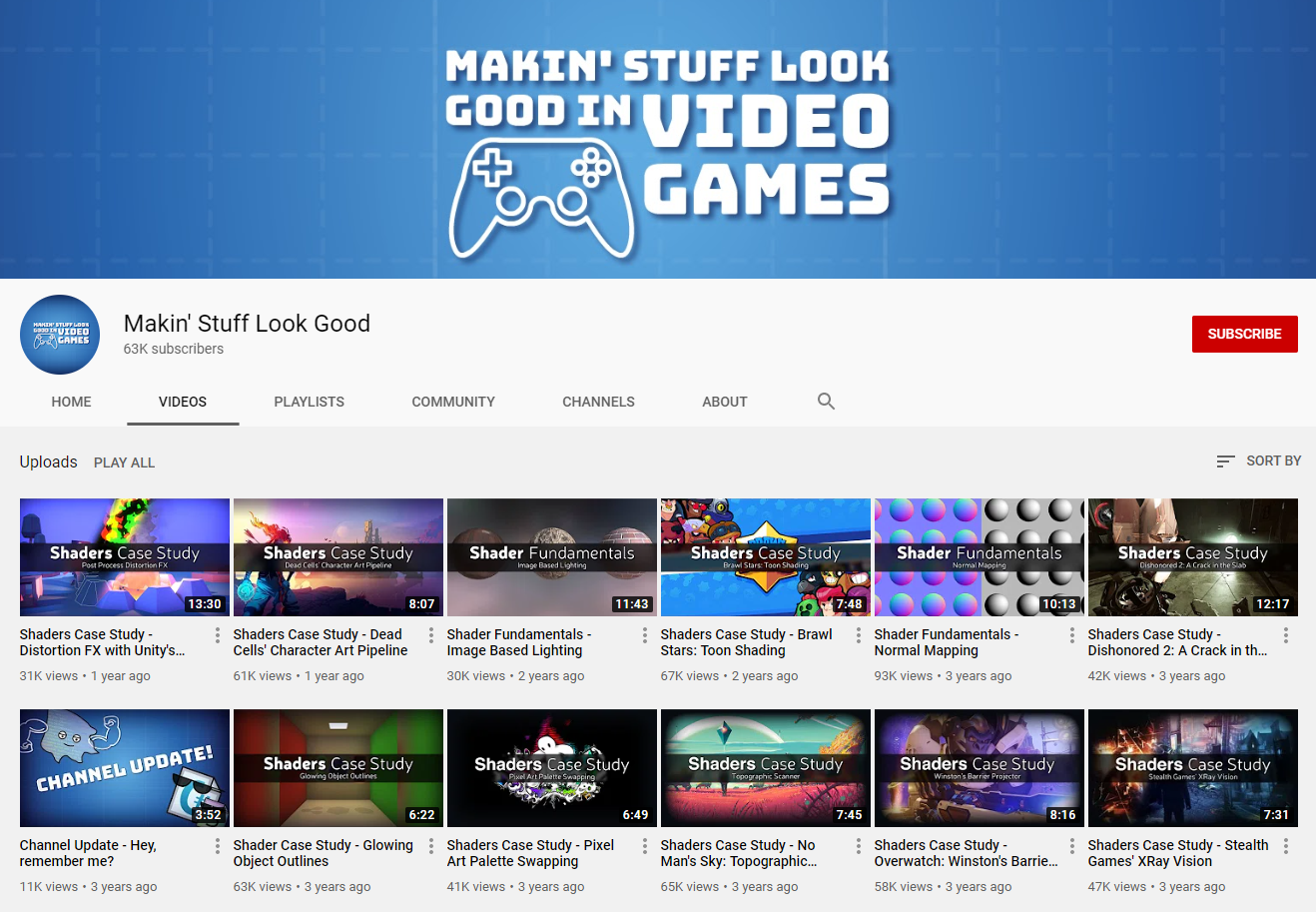### Homepage Description for the "Macon's Stuff Look Good" Website

The homepage features a striking blue background that transitions from dark blue on the left to a lighter blue in the center, and back to a darker blue on the right. In the center of this background, bold white text prominently displays the channel's name and tagline:

**Middle Text:**
- "Macon's Stuff Look Good"
  - "Video Games" (in larger, bold lettering)

Below the tagline, there is an outlined white image of a PlayStation controller nestled under the word "Good."

### Main Section
Following this, the page transitions to a white background. In the top-left corner, a circular icon contains the text:
- "Macon's Stuff Look Good"
- "63K Subscribers" (both in black)

To the right of this circular icon, bold black text states "Macon's Stuff Look Good."

Adjacent to this section, there is a prominent red tab with the word "SUBSCRIBE" in all capital letters, urging visitors to join the community.

### Navigation Bar
On the left side of the white background, a navigation menu lists:
- **Home** (in black, all caps)
- **Videos** (underlined in black)
- **Playlists, Communities, Channels, About** (each in black)
- A search icon is also present.

### Content Display
Below the navigation bar:
- The left section begins with "Uploads" and a "Play All" option.
- The right section features a "Sort By" dropdown menu with an icon.

Further down, six featured videos are displayed in a two-row grid. Each video displays:
- The thumbnail image
- The video's name across the middle of the thumbnail
- The video's duration in the bottom-left corner of the thumbnail

Below each thumbnail:
- Additional information about the video
- The number of views
- The date it was posted